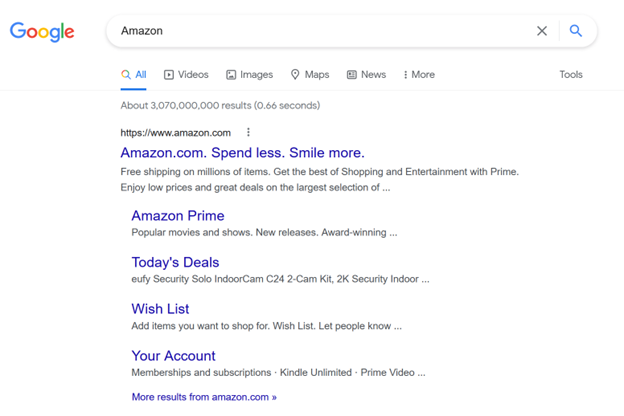This is a screenshot of a Google search results page. In the top-left corner, the multicolored Google logo is displayed, with the letters colored as follows: the first 'G' is blue, the first 'O' is red, the second 'O' is yellow, the second 'G' is blue, the 'L' is green, and the 'E' is red. 

To the right of the logo, the search bar contains the query "Amazon." Below the search bar, a grey navigation menu lists search categories: "All," "Videos," "Images," "Maps," "News," "More," and "Tools." The "All" category is highlighted in blue, indicating it is the active filter.

The first search result is for Amazon.com. The clickable URL "https://www.amazon.com" is displayed, followed by a brief description: "Amazon.com, spend less, smile more. Free shipping on millions of items. Get the best of shopping and entertainment with Prime. Enjoy low prices and great deals on the largest selection of..." with the rest truncated by an ellipsis.

Underneath, another clickable link labeled "Amazon Prime" appears in blue, accompanied by a description: "Popular movies and shows, new releases, award-winning..." followed by an ellipsis.

Further down, a blue link titled "Today's Deals" is present. Its description in grey reads: "Eufy Security Solo Indoor Cam C24 2 Cam Kit, 2K Security Indoor..." truncated by an ellipsis.

The next blue link says "Wishlist," with a grey description beneath it: "Add items you want to shop for, Wishlist, let people know..."

Finally, the last blue link reads "Your Account." The supporting text indicates various sections: "Memberships and Subscriptions, Kindle Unlimited, Prime Video," and at the very bottom, "More results from Amazon.com" followed by two right-facing arrows.

This detailed caption captures the various elements and textual information displayed in the Google search results for "Amazon," providing a comprehensive overview of the screenshot.